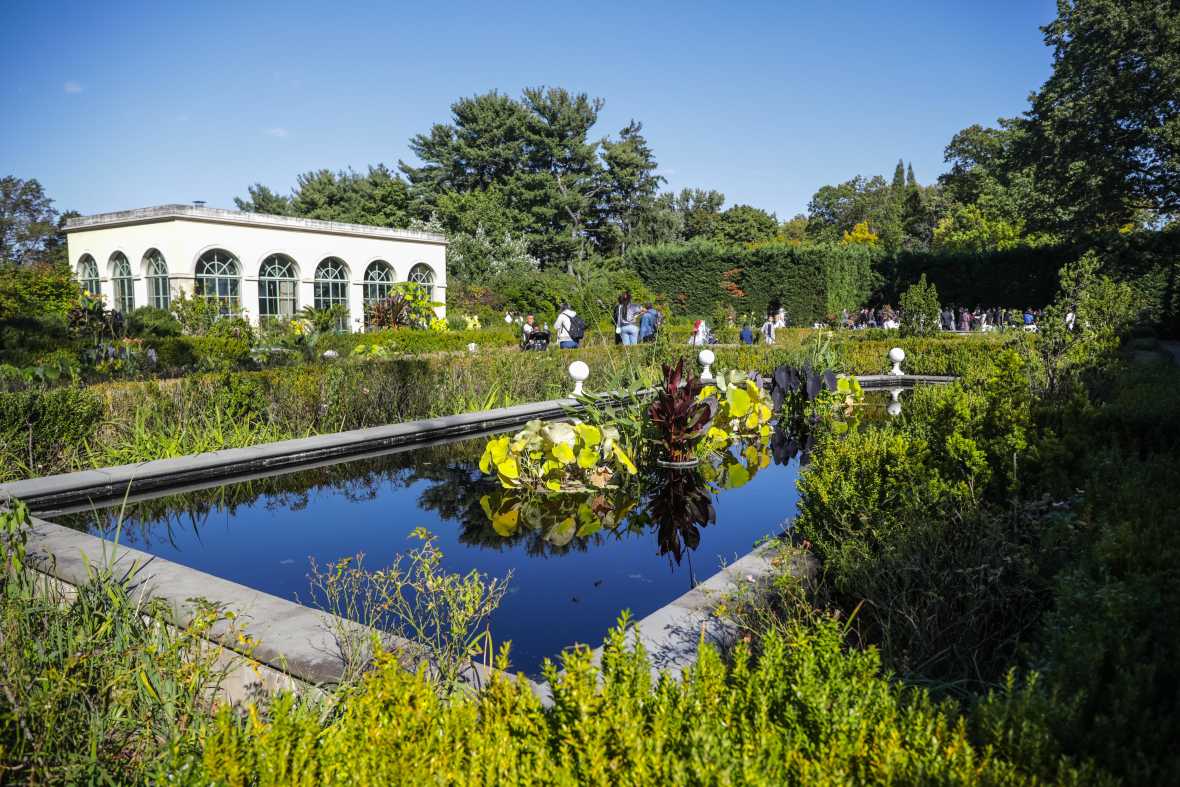The photograph captures a meticulously manicured garden nestled within a lush forest, brimming with greenery. Dominating the foreground is a rectangular man-made pool, teeming with well-maintained lily pads, three or four of which tower majestically above the water. One lily pad features a striking purple hue, while the others are a vibrant green. Encircling the pool are an array of verdant plants and topiaries, adding to the garden's allure. In the distance, a stately white building with rounded windows replete with iron bars stands prominently, possibly serving as a conservatory. The scene is alive with activity, as people mill about, suggesting a garden party atmosphere. The sky above is a clear, light blue with a few wisps of white clouds, indicating beautiful, warm weather. Many attendees are donning hats to shield themselves from the sun as they stroll through the picturesque grounds. The background is dominated by a variety of green trees and tall hedges, creating a secluded and serene courtyard feel.